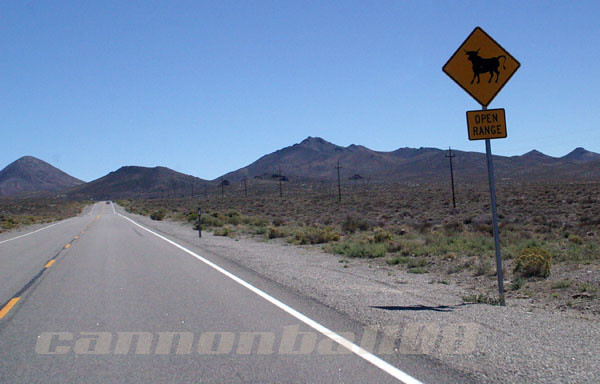The photograph depicts a desolate two-lane highway cutting through a barren, arid landscape with a backdrop of a mountain range extending horizontally across the middle of the image. The sky is a clear, vivid blue with no clouds in sight. On the right side of the road, there's a silver pole featuring a yellow diamond-shaped sign with a black silhouette of a cow, accompanied below by a rectangular yellow sign that reads "Open Range" in black text. Power lines can be seen running parallel to the road, stretching back towards the imposing mountains. The terrain around the road is devoid of trees and buildings, consisting mainly of flat, sandy areas with sparse patches of scrub grass. Additionally, a faint glimpse of a car can be seen far in the distance, adding to the sense of isolation. At the bottom of the image, there's a watermark that reads "Cannonball 08," which subtly overlays the photograph.